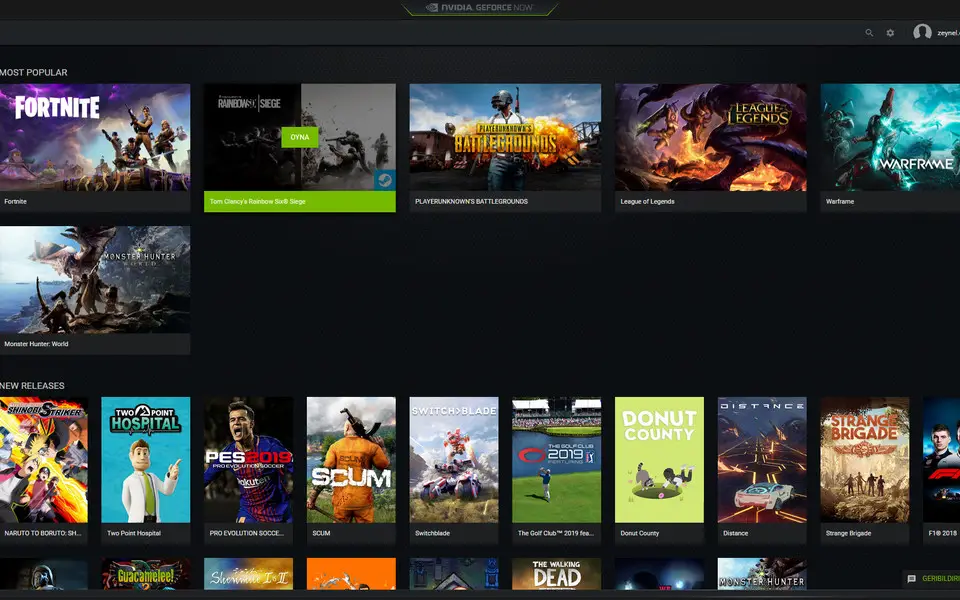The image depicts a screenshot of the NVIDIA GeForce Now game launcher application, showcasing its clean and user-friendly interface. The app features a dark mode theme with a black and dark gray color scheme. 

At the top of the interface, there is a prominent banner with a green outline displaying the NVIDIA GeForce Now logo alongside the NVIDIA emblem. Situated just below this banner, the navigation area contains a search bar, a cogwheel icon for settings, and a profile icon.

Directly beneath the navigation area, there is a "Most Popular" section, highlighting the top games with vivid thumbnails. Featured in this section are popular titles such as Fortnite, Rainbow Six Siege, PlayerUnknown's Battlegrounds, League of Legends, Warframe, and Monster Hunter: World.

Following the "Most Popular" section, a "New Releases" category showcases fresh game arrivals, each represented by a thumbnail. The newly added games include Naruto to Boruto, Two Point Hospital, PES 2019, Scum, Switchblade, The Golf Club 2019, Donut County, Distance, and Strange Brigade.

Overall, the image captures the comprehensive layout and design of the NVIDIA GeForce Now storefront, highlighting its streaming service capabilities and diverse game offerings.